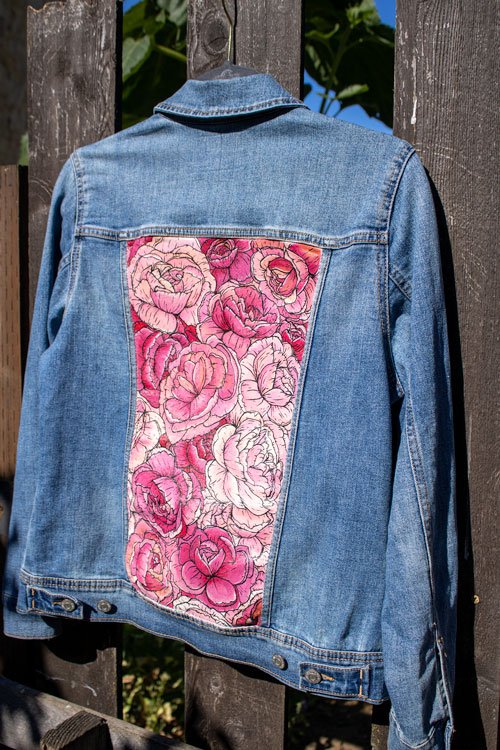A light to medium denim jacket hangs on a dark wooden fence, its material faded from wear and sun exposure. The fence, constructed of dark gray wood streaked with white, stands under a bright, sunny sky, with glimpses of greenery—trees and bushes—visible through its slats and at its base. The jacket, displayed from the back, reveals intricate embroidery in its central panel, stretching from the bottom of the shoulders to the waist. The embroidery is an elaborate bouquet of roses in shades of pink and red, outlined in black to highlight the detailed petals. The jacket rests on a hanger, accentuating the sunny outdoor setting, with small buttons visible at the front.